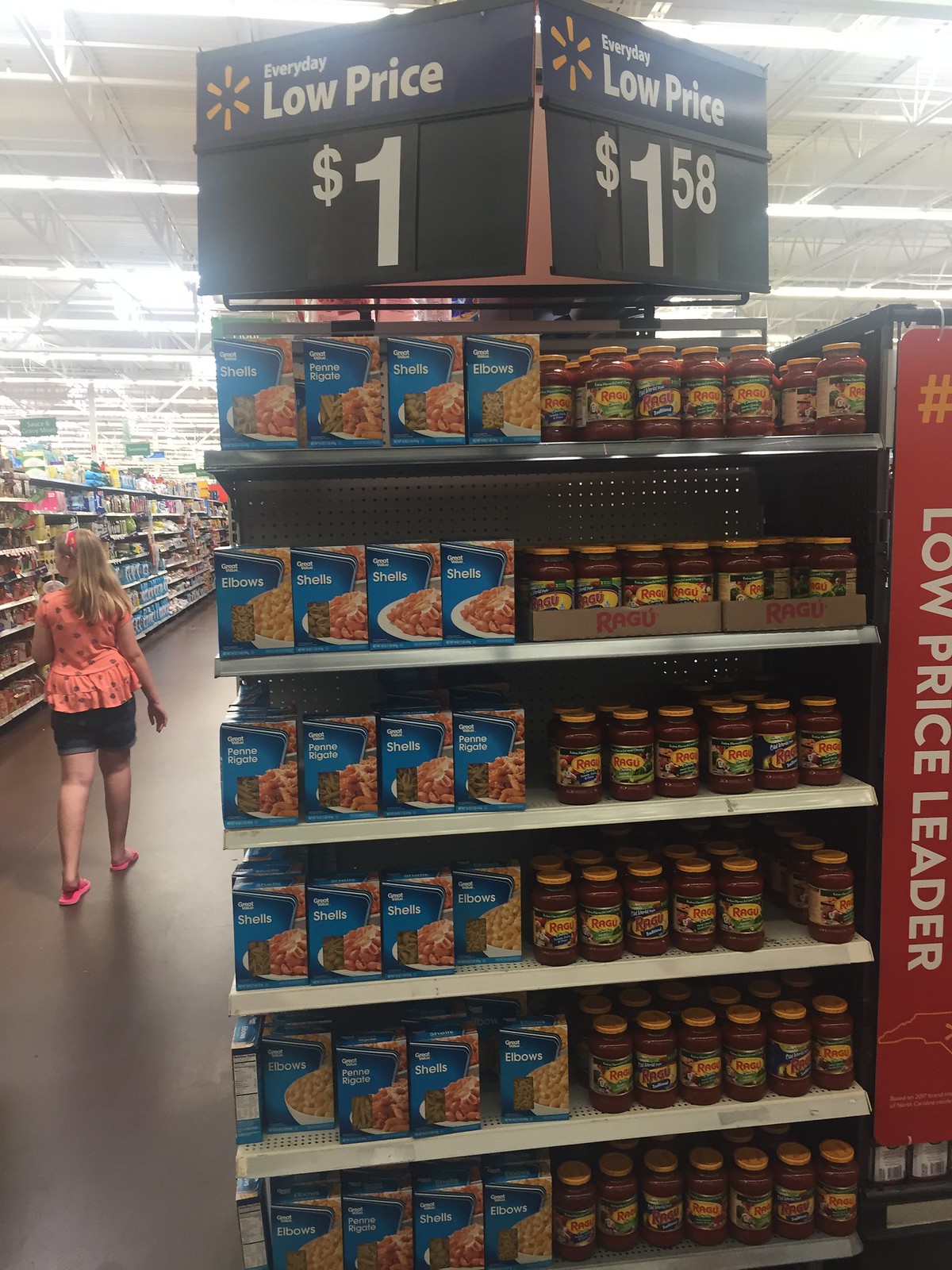The image depicts the interior of a Walmart store, specifically focusing on a food section featuring prominent black price tags. The signs, bearing the Walmart symbol, advertise "Everyday Low Price" offers. One sign indicates a price of $1 for what appears to be boxed food items, possibly a type of noodles or other packaged goods. Another sign lists a price of $1.58 for Ragu pasta sauce. In the left portion of the image, a Caucasian woman with blonde hair is visible. She is dressed in a printed pink, very short-sleeve blouse and blue jean shorts, along with pink flip-flops. The woman is walking down the aisle, partially facing away from the camera.